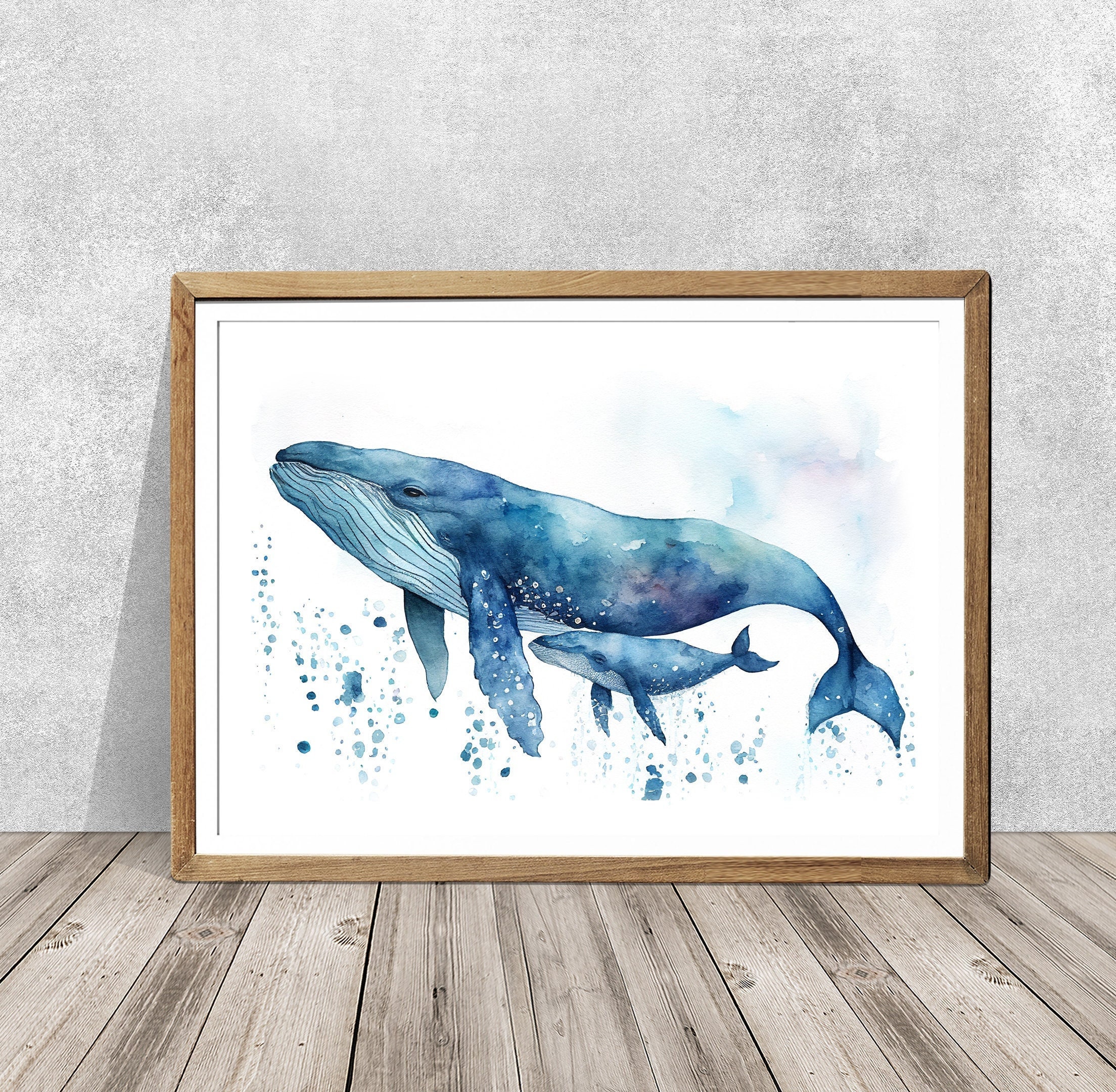This image showcases a watercolor painting encased in a slim, honey-brown wooden frame with white matting. The painting, which appears to be resting against a gray speckled wall on a shabby chic wooden floor, depicts two blue whales — a fully grown adult and a small baby, suggesting a mother and calf. The mother whale is predominantly blue with a distinctive white belly lined with vertical grooves, while the baby whale, just a few months old, also features blue and white hues. Both whales are depicted swimming leisurely, accompanied by splotches of blue and purplish paint that likely represent bubbles rising beneath them. The overall background of the painting is primarily white with subtle hints of bluish and purplish tones.